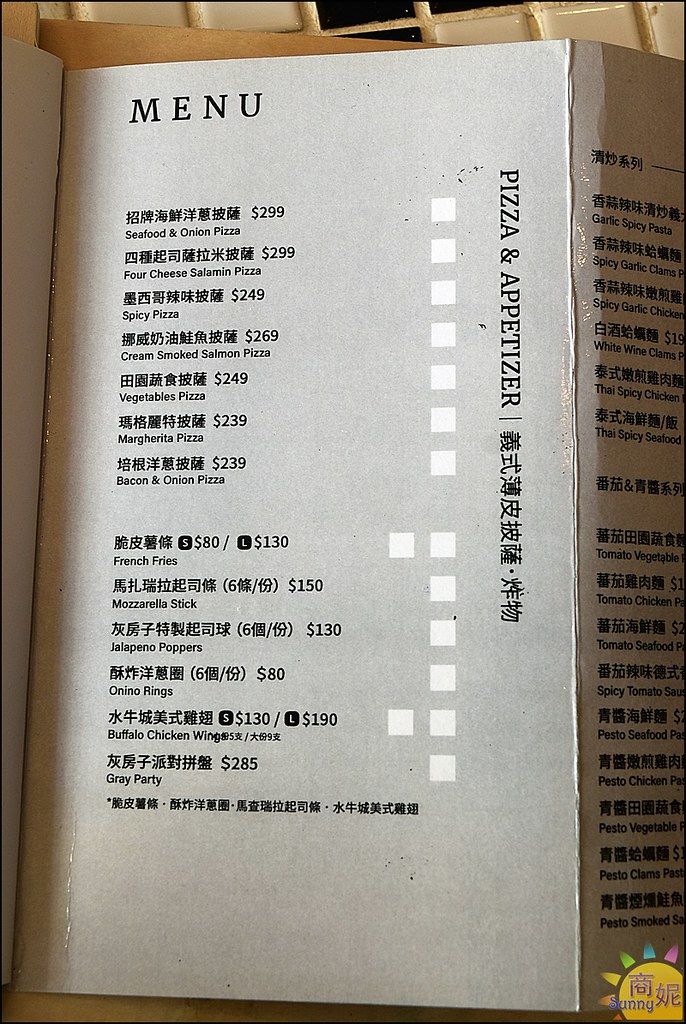The image showcases a menu with a clean white background. Prominently displayed at the top is the word "MENU" in black text. Beneath this, there is a section adorned with intricate Chinese calligraphy. Following this, the menu lists several food items in both English and Chinese, along with their corresponding prices.

In the first section, we observe:
- Seafood and Onion Pizza priced at $2.99
- Vegetable Pizza for $2.49
- Margarita Pizza at $2.39
- Bacon and Onion Pizza for $2.39

After a small gap of a couple of inches, the menu continues with:
- French Fries priced at $1.30
- Mozzarella Sticks for $1.50
- Jalapeno Poppers at $1.30
- Onion Rings for $0.80
- Buffalo Chicken Wings at $1.90
- Gray Party for $2.85

The lower portion of the menu features a vertical arrangement of white squares. Below these, in black text, the words "Pizza and Appetizer" are displayed, followed by a straight line and more Chinese writing.

On the right side of the menu, only part of the text is visible, and it is quite small. Near the bottom, we can make out words such as "tomato," "seafood," and "pesto chicken." In the lower right corner, there is a vibrant image of a sun with short rays in shades of green, blue, and pink radiating outward.